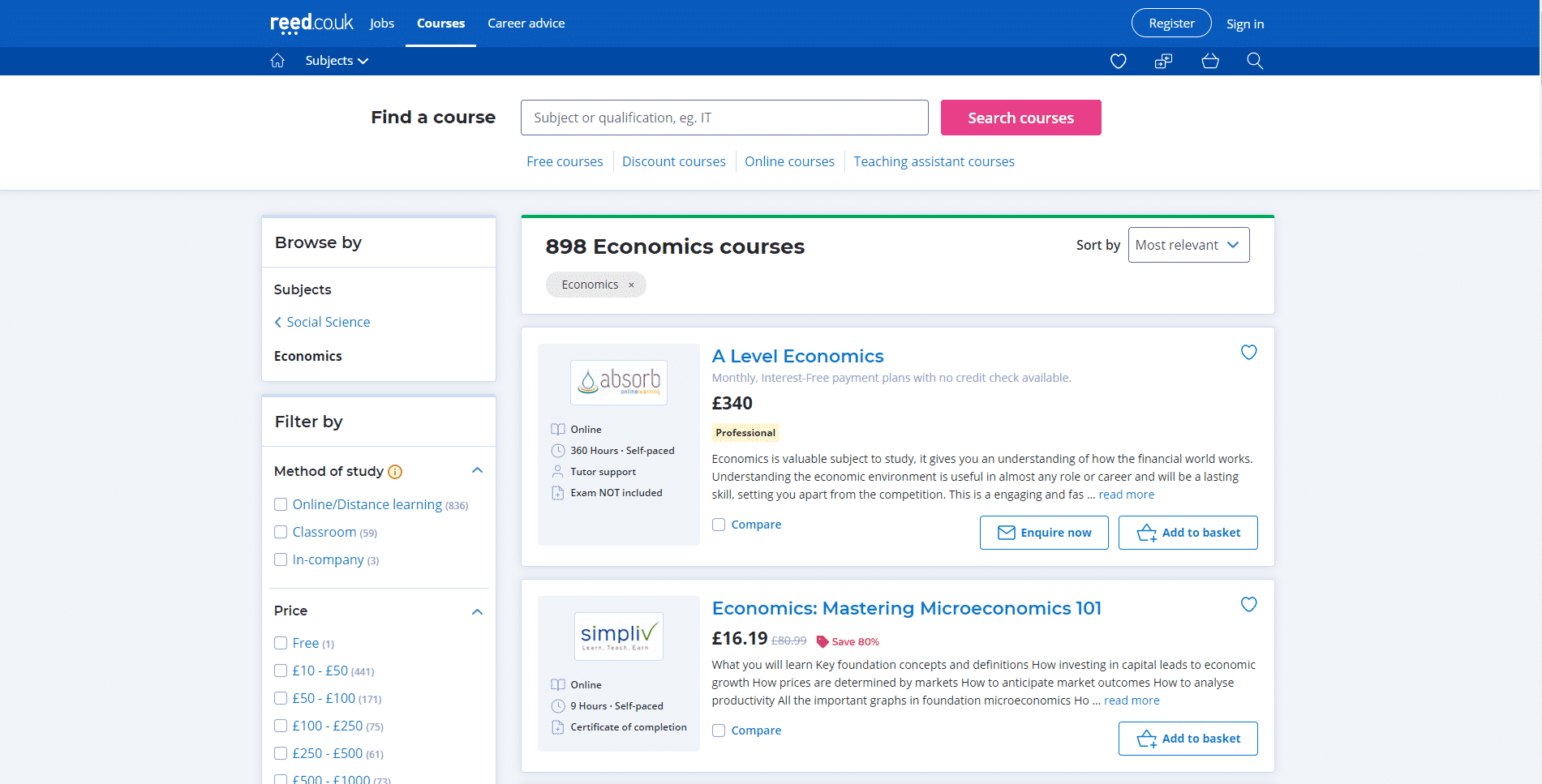The web page from readco.uk is designed to provide a user-friendly interface for job seekers, learners, and career planners. At the very top, there is a prominent blue box displaying the site name "readco.uk" alongside navigation options labeled "Jobs," "Courses," and "Career Advice." The "Courses" option is highlighted with a white underline, indicating it is the current selection. Situated on the left, this section is balanced on the right by buttons for "Register" and "Sign In."

Immediately below, a darker blue banner houses navigational icons and options. On the left, a house icon serves as the home button, next to which "Subjects" is listed with a downward arrow indicating a dropdown menu. On the right-hand side, users will find icons for favorites, comparison (two arrows and boxes), a shopping cart, and a search magnifying glass.

Directly beneath this banner, the page features a prominent message, inviting users to "Find a Course," accompanied by a search bar and a button labeled "Search Courses."

The main body of the page is organized into three columns. On the top left, a white text box includes options to "Browse by Subjects," specifically listing "Social Science" and "Economics." Below this, users can "Filter by" criteria such as "Method of Study" and "Price."

In the center of the page, another white text box announces "898 Economics courses," with a dropdown menu set to "Sort by: Most Relevant." The first two courses listed are "A Level Economics" and "Economics: Mastering Microeconomics 101."

This well-structured layout ensures that visitors can easily navigate and access the multitude of educational resources available.